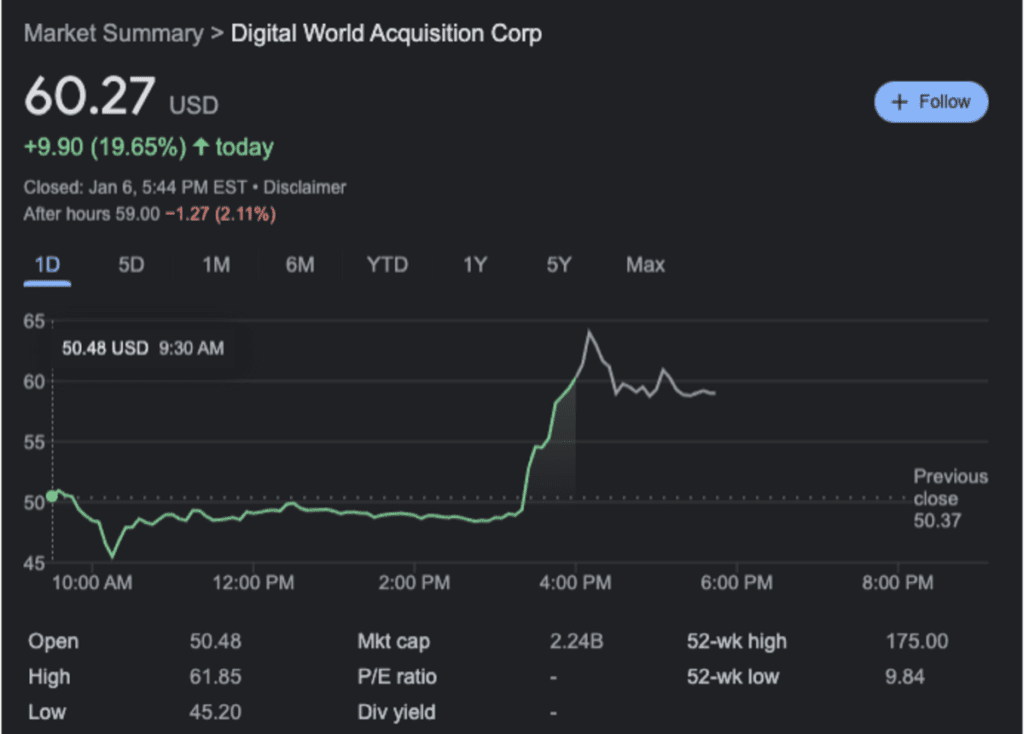Screenshot Description:

The image is a screenshot with a black background, titled "Market Summary" in gray font located in the upper left corner. An arrow points to the stock title "Digital World Acquisition Corp." Below this, the stock price is listed as "$60.27 USD," showing a gain of "$9.90" which constitutes a 19.65% increase for the day. The closing time is marked as "January 6th at 5:44 p.m. EST" with a note about a disclaimer next to it. Following the closing information, it mentions that the price has dropped by "$1.27" or 2.11% to $59.00 as of the time of the screenshot.

To the right, there is a light blue "Follow" button featuring a plus symbol, allowing users to track the stock.

Below these details is a chart displaying the stock's performance throughout the day with the price range between $45 and $65. Time intervals are marked at 10 a.m., 12 p.m., 2 p.m., 4 p.m., and market close at 6 p.m. The graph indicates a sharp increase, peaking above $60.27 before a downward trend as the market closed.

Additional data available includes the opening price, high and low prices of the day, market capitalization, and the stock's 52-week high and low, offering a comprehensive context for the stock's performance.